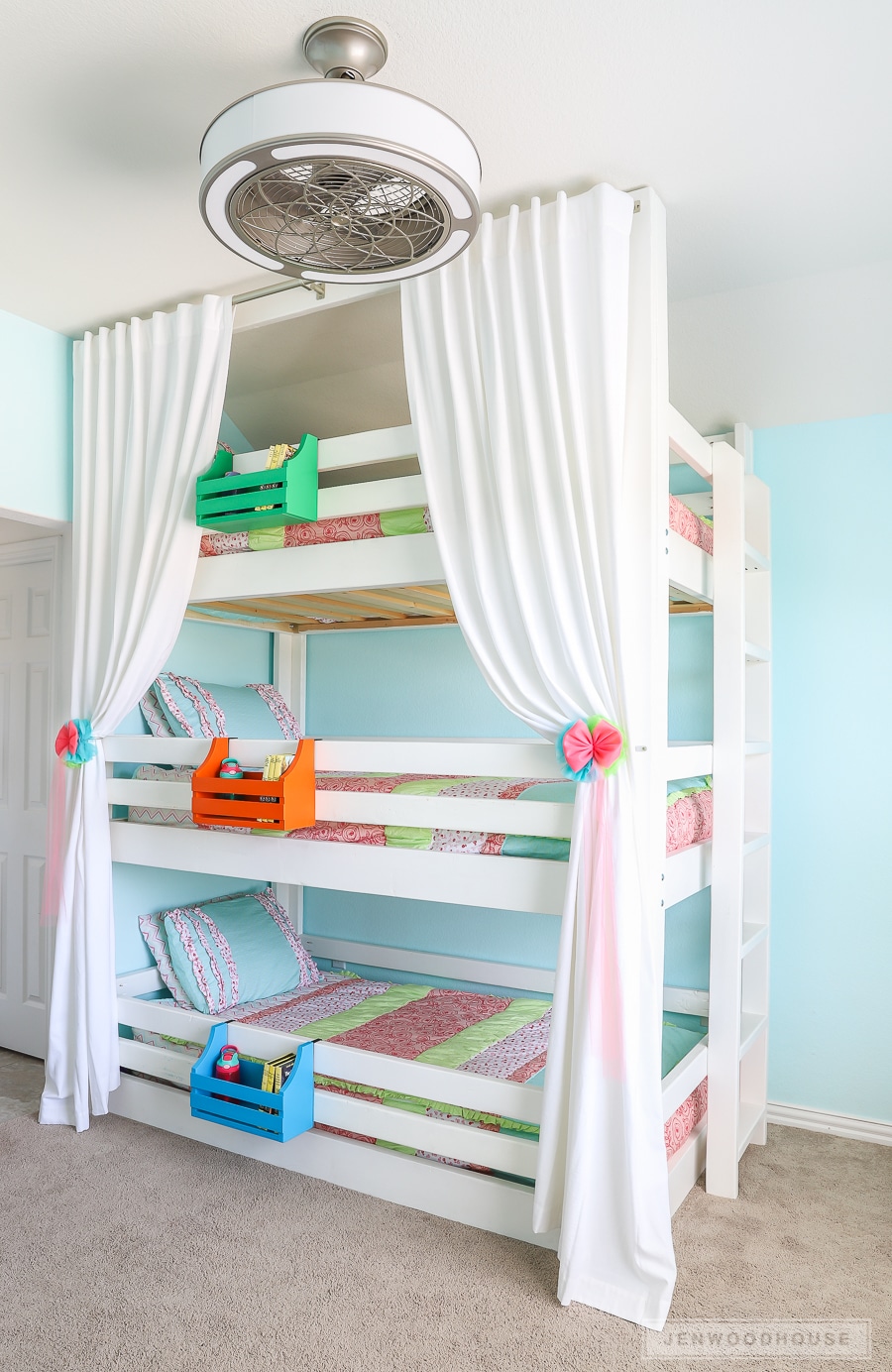This image captures a cozy, sky-blue themed bedroom with a unique triple bunk bed setup, likely designed for children. The walls are painted a serene, beachy light blue, reminiscent of a clear sunny day, while the ceiling and doors are a crisp white. The cream-colored carpet adds warmth to the room. 

Dominating the center of the space is the striking triple bunk bed, constructed with white slat boards and featuring three stacked twin-sized beds. These beds are adorned with charming quilts in varying colors including pink, green, and blue, which harmonize beautifully with the room’s color scheme. Each bed has matching blue pillows edged with pink and white ruffles. 

For added privacy and charm, long white curtains are attached to the bed frame, elegantly tied back with pastel bows in shades of pink, blue, and yellow. At each level of the bunk bed, a small, painted caddy hangs from a rail, each in different colors—green for the top bunk, orange for the middle, and blue for the bottom. These caddies hold an array of items such as books and toys, with one appearing to contain a water bottle. 

Additional details include a glimpse of a white closet door on the left and the watermark "Jen Woodhouse" at the bottom of the photo, indicating the original source. The neatly arranged elements and thoughtful touches suggest this is a well-loved space tailored for comfort and functionality.